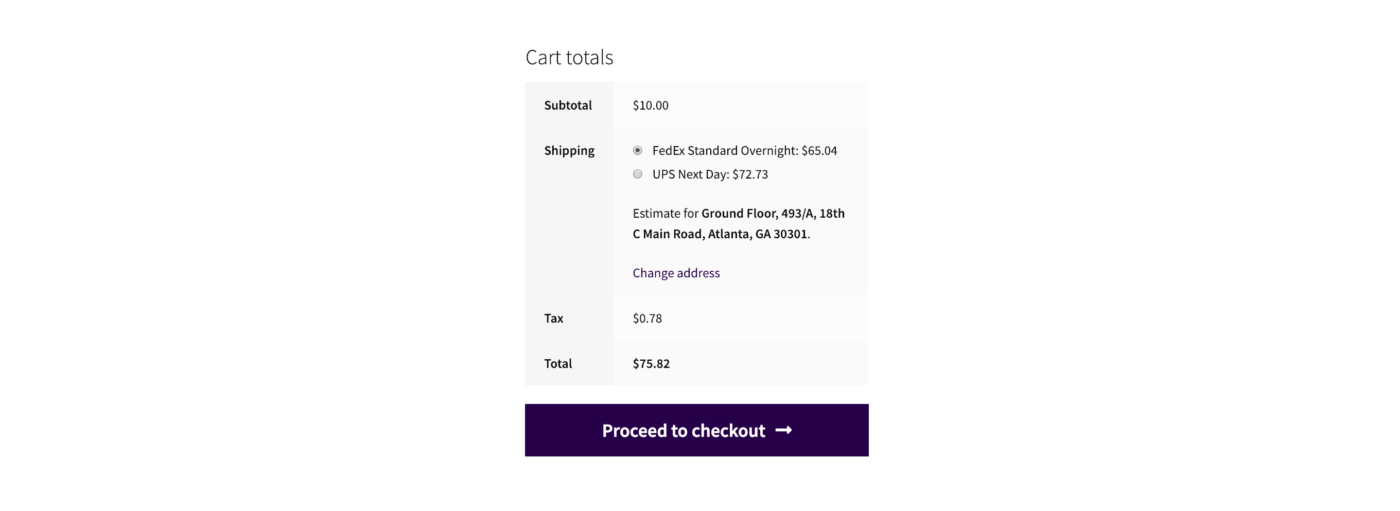The image displays a detailed summary of a cart checkout screen. At the top left, there's a bold, black text that reads "Cart Total" against a white background. Below this, "Subtotal" is listed with an amount of $10.00. 

The shipping section offers two options: "FedEx Overnight" at $65.04, which is the selected option, and "UPS Next Day" at $72.73. Further down, the address for the shipping estimate is displayed as "Ground Floor 493/A, 18th C, Main Road, Atlanta, GA 30301", accompanied by a purple text link that says "Change Address."

On the left, there's a text that reads "Tax" with a corresponding amount of $0.78. At the bottom, the "Total" price is calculated as $75.82, summing up the subtotal, shipping cost, and tax.

Finally, at the very bottom, there's a prominent, purple button with white text that urges the user to "Proceed to Checkout."